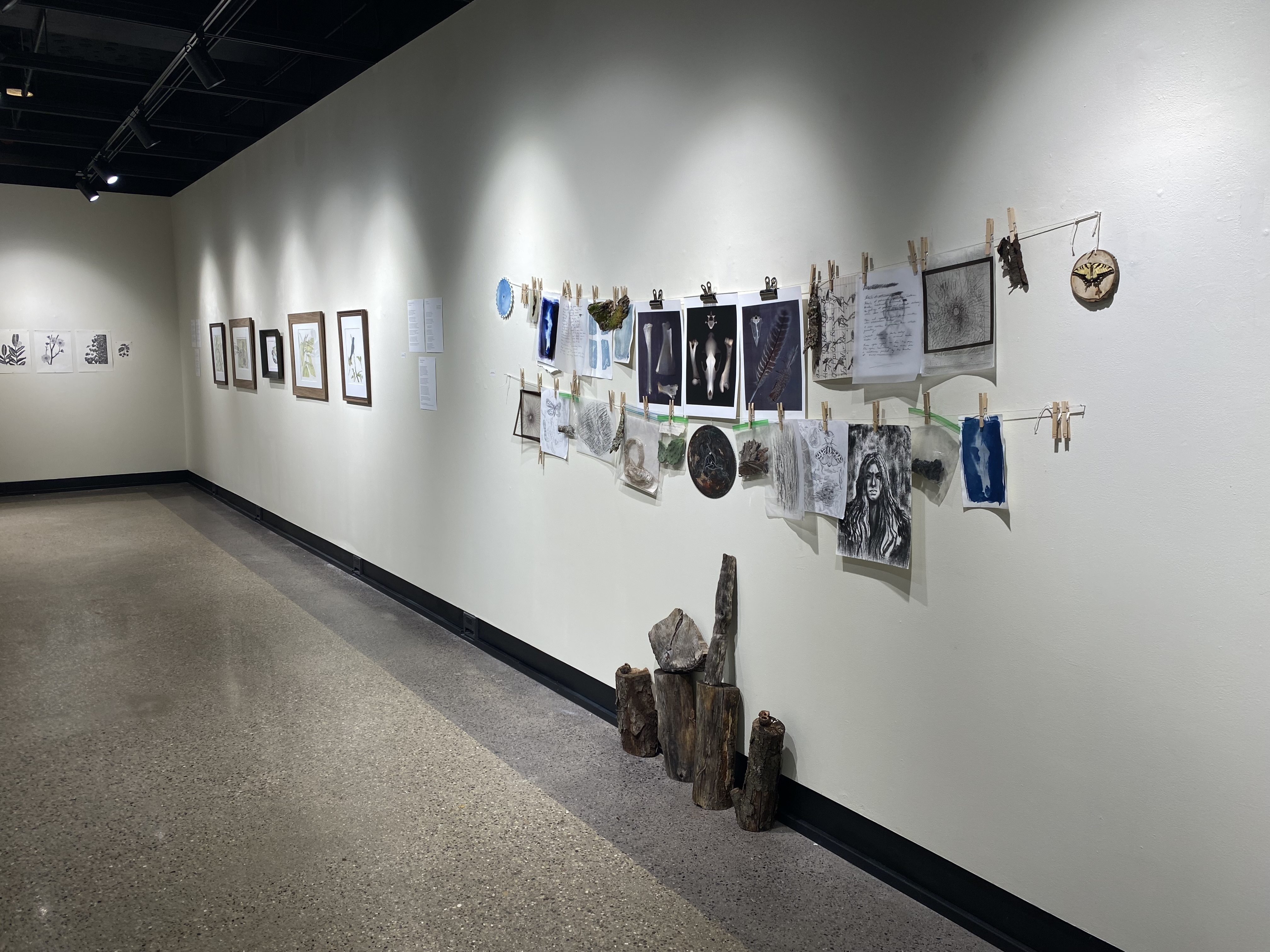The image depicts the interior of what appears to be either a university sociology office or an art gallery. The focal point is a clothesline stretched from one wall to the other, displaying various artworks and drawings held up by clothespins. The artworks include a photograph of a woman, a horse skull, candle illustrations, and a bearded man. Below the clothesline are four logs of firewood, with the logs on either end topped with rocks and the middle ones topped with another log and a large rock respectively.

The walls are painted white, creating a bright and neutral backdrop, illuminated by white lighting. The floor is polished cement, adding a sleek and modern touch to the space. Along the longest wall, five framed pictures are displayed, though their subjects are difficult to discern. There are three more pieces of paper taped to the wall closer to the viewer. Additional unframed pictures are seen on the back wall, contributing to the eclectic and creative atmosphere of the space.